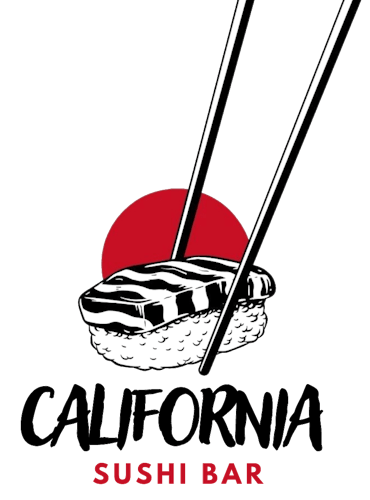The image is a stylized, digitally-drawn logo for a restaurant called "California Sushi Bar," set against a predominantly white background. At the center of the image is a vibrant red circle, reminiscent of the Japanese rising sun, symbolizing the theme of the restaurant. Superimposed over the red circle is an intricately drawn piece of sushi, with detailed black-and-white marbleized meat on top of rice. Two black-and-white chopsticks are depicted coming in from the top right of the image, poised to pick up the sushi. Beneath the sushi illustration, the restaurant name is displayed: "California" in large black graffiti-style block letters, and "Sushi Bar" in smaller red text underneath. The overall color palette consists of white, black, red, and gray, emphasizing the Japanese-inspired aesthetic of the logo.